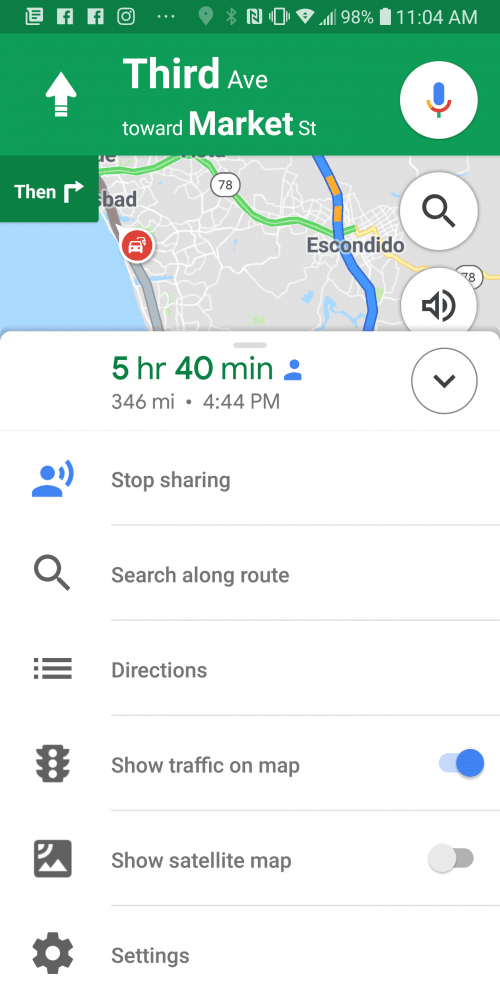The image is a screenshot with a white background displaying navigation information. At the top of the screen, there is a directional prompt indicating "3rd Avenue toward Market Street" with an upward and right-pointing arrow. Below this prompt, a series of circular icons are arranged: a white circle with a microphone icon in Google colors, a white circle with a magnifying glass, and another circle with a speaker icon.

In the upper right corner, the status indicators show the battery at 98%, the time at 11:04 AM, and the Bluetooth symbol. The map itself indicates a route covering 346 miles, with an estimated duration of 5 hours and 40 minutes, and an expected arrival time at 4:44 PM. There is also a blue profile icon for user identification and a blue icon featuring a person with two lines, suggesting voice interaction options.

Below the map, there are various functional buttons and options. The "Stop Sharing" button is visible, alongside the "Search Along Route" button with a magnifying glass icon. The "Directions" button is symbolized with three rectangles. The "Show Traffic on Map" option is toggled on, indicated by the associated traffic light icon. The "Show Satellite Map" option has the toggle bar turned off.